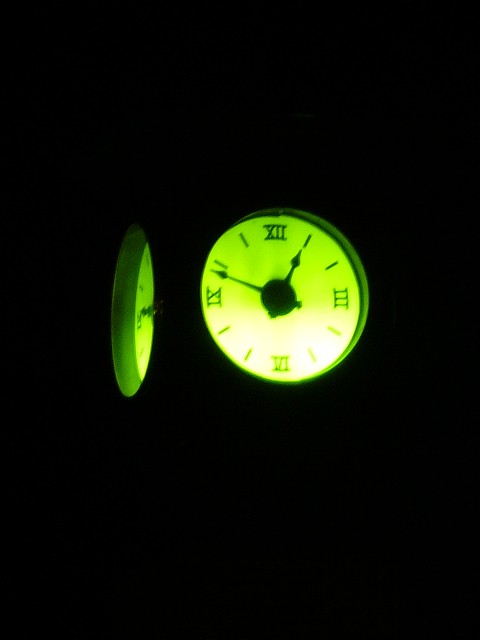This image is a nighttime photograph featuring two illuminated clock faces against a pitch-black background. The central focus is a clock with a circular face backlit in bright green, displaying Roman numerals for the hours 3, 6, 9, and 12, while the remaining hours are marked by simple black dashes. The clock hands show a time of 12:50, with the shorter hand pointing at the 1 and the longer hand at the 10. Additionally, this clock is accentuated with a white light emitting from its bottom. Just to the left, another clock with a similar design is partially visible, adding depth and symmetry to the image. The overall effect is striking, capturing the glow of the clocks against the void of the night sky.